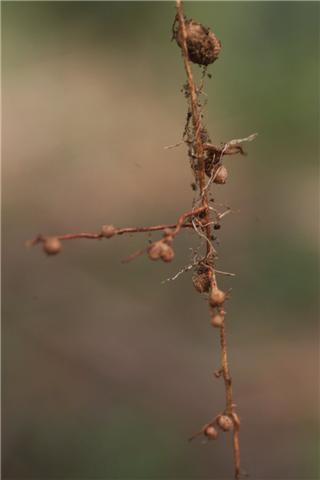The image showcases a close-up view of a very thin, twig-like branch with a dense, string-like vine wrapped around it. The branch forms a T-shape, with the main section extending vertically and another piece jutting out at a 90-degree angle toward the left side of the frame. Adorning the branch are numerous small, brown, spherical objects that resemble tiny berries or seeds, with a larger one positioned near the top. The background is heavily blurred, exhibiting a shallow depth of field, and features a mix of green, tan, and light pink hues, contributing to an overall muted backdrop that contrasts with the detailed subject.